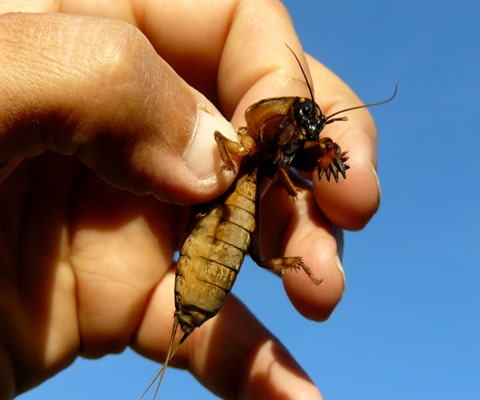A detailed caption for the image could be:

In this image, a light brown-skinned hand, entering from the left side, is delicately pinching a large insect between the thumb and pointer finger. The insect, resembling a mix between a cockroach and a cricket, takes center stage in the photo. The insect's head is black with two wavy, black antennas. It has spiky legs that are a mix of brown and black, along with a translucent brown back and a light tan or yellowish belly. The abdomen, which looks like a massive egg sac and makes up about 60% of its length, is lighter brown. Two small, translucent tan tails protrude from the bug's rear. The background to the right of the insect is a clear blue sky, enhancing the colors of both the hand and the insect. It's unclear whether the person is posing with the insect or handling it for research purposes.